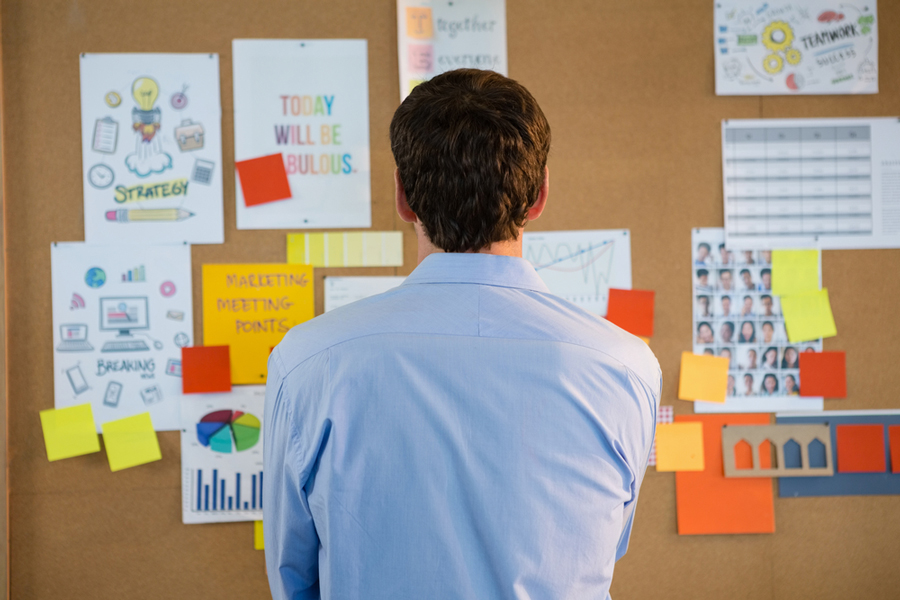The photograph shows the back of a young man with short dark hair, wearing a clean light blue long-sleeve dress shirt. He stands facing a bulletin board, which is brown in color. The board is cluttered with various items, including white sheets of paper containing crayon drawings, some of which appear to have been made by children. The board also features several sticky notes, a pie chart in red, blue, green, and yellow, and additional blank orange and blue sheets of paper. To the left of the board, there are notes with messages like "today will be fabulous" and "strategic strategy," along with a section labeled "marketing meeting points." Photos of faces are attached to the right side of the board. The scene conveys a sense of contemplation or planning, possibly within a professional setting.